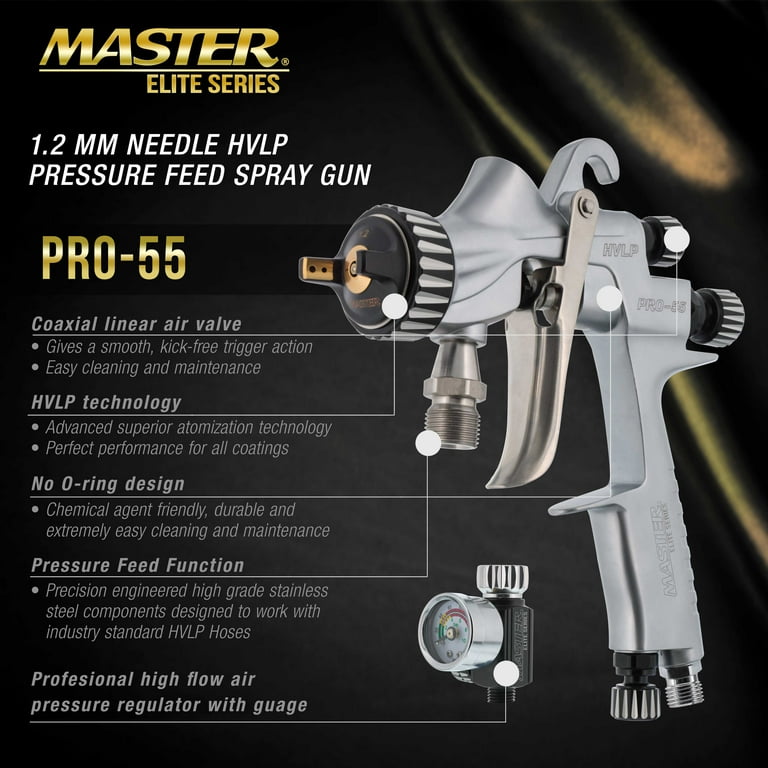This striking advertisement showcases the sophisticated Master Elite Series 1.2 millimeter needle HVLP pressure feed spray gun, Pro 55. Set against a sleek black background with a subtle ripple effect in the upper right corner reminiscent of a curtain, the image exudes a sense of premium quality and precision. The focal point on the right side is the spray gun itself, an elegant silver tool with metallic accents and an ergonomic design. It features a functional nozzle, a smooth metal trigger, and various fittings for versatile connectivity. Important components like the professional high-flow air pressure regulator with a gauge are highlighted, providing a clear close-up view.

On the left, the advertisement is topped with the title "Master Elite Series" in striking gold text, followed by the product description: "1.2 millimeter needle HVLP pressure feed spray gun." The model name "Pro 55" is also emphasized in gold text. Below this, a series of bullet points delineate the spray gun's advanced features: a coaxial linear air valve for a smooth, kick-free trigger action, superior HVLP technology for advanced atomization, a no O-ring design for enhanced durability and chemical resistance, and high-grade stainless steel components for precision performance with standard HVLP hoses. Each feature is linked with lines pointing to specific parts of the spray gun, making the ad both informative and visually engaging.